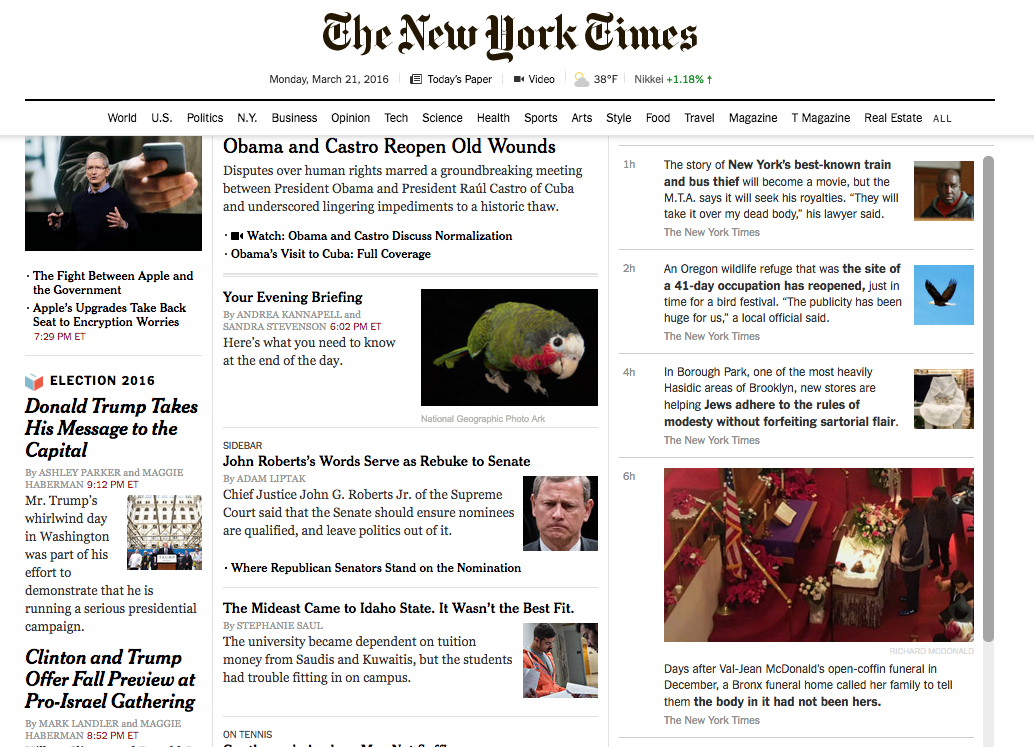Screenshot of The New York Times homepage, dated Monday, March 21st, 2016, indicating an online edition. The top banner shows options for accessing today's paper and video content. Current temperature is displayed as 38 degrees Fahrenheit, and the Nikkei index shows a positive change of +1.18%. Below the masthead, there are clickable sections for World, U.S., Politics, New York, Business, Opinion, Tech, Science, Health, Sports, Arts, Style, Food, Travel, Magazine, T Magazine, and Real Estate, with an option to view all sections.

The left column features prominent headlines such as "The Fight Between Apple and the Government," "Election 2016: Donald Trump Takes His Message to the Capitol," and "Clinton and Trump Offer Fall Preview at Pro-Israel Gathering." The middle column highlights stories like "Obama and Castro Reopen Old Wounds," "Your Evening Briefing" which is paired with an image of a tropical bird, "John Roberts' Words Serve as a Rebuke to the Senate," and "The Middle East Came to Idaho State: It Wasn't the Best Fit." Additional articles of local or state interest line the right side of the page.